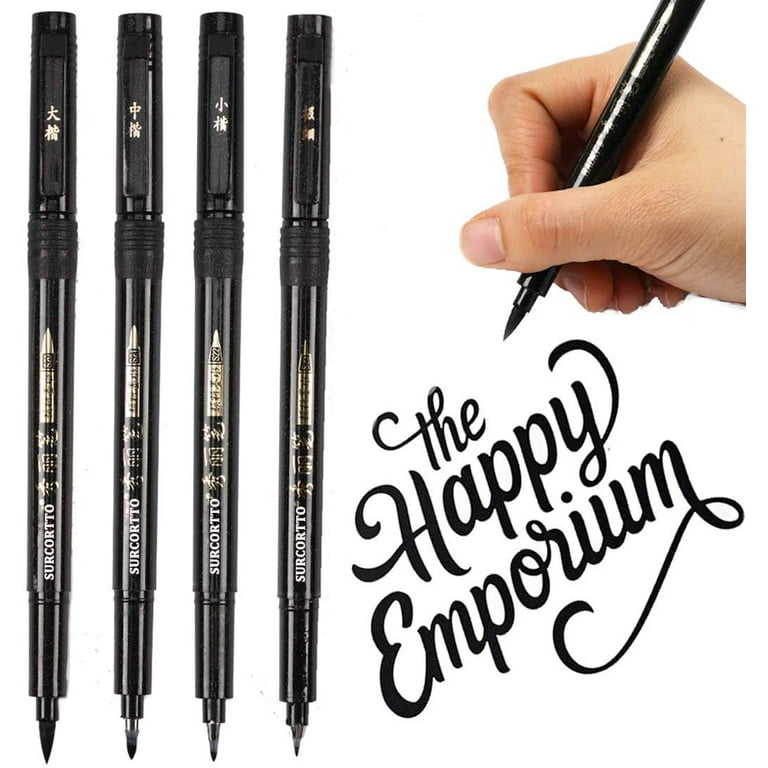The image is a minimalist advertisement set against a white background, showcasing a collection of pens from "The Happy Emporium." On the left side of the image, four pens stand vertically, with tips exposed, presenting different sizes for varied line thickness ranging from thick to thin. Each pen features cylindrical bodies with pointy ends and clips adorned with Chinese characters. The focal point to the top right shows a hand grasping one of these black thick pens, poised to write. Below this, angled at a 45-degree slant, is the brand name "The Happy Emporium" elegantly written in bold cursive, suggesting that the pens are likely designed for calligraphy or fine writing.